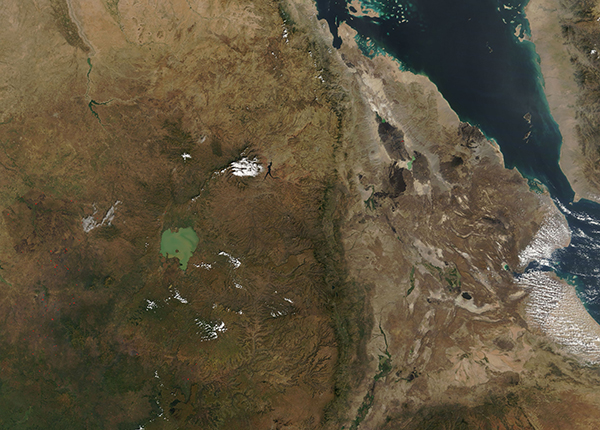This is a satellite image providing a high-altitude, horizontally-aligned view of a region that predominantly features various shades of brown land, with the darkest shades concentrated in the middle and lower left sections. The central part of the darkest area contains a small, vivid green section, surrounded by several white spots, possibly indicating clouds or snow cover on the mountains. As the image extends to the upper right, the brown land transitions to a lighter hue before being intersected by a narrow stretch of dark bluish-gray water likely representing a part of the Red Sea. The top right corner showcases this water body with a narrow opening. The landscape depicted appears largely uninhabited, characterized by mountains, plains, and deserts, with no visible cities. The overall scene includes unique land formations and a blending of green, brown, blue, and white tones, capturing a detailed and diverse piece of the Earth's surface.